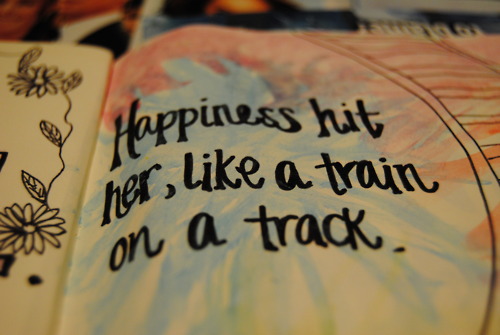This is a close-up image of a notebook or possibly a quilt-like fabric featuring a prominent saying. The background consists of a white, quilted or fabric texture with various artistic elements. On the right side, there is a light blue flower with red floral shading above it, which could suggest watercolor or light marker. In the very center of this page, large, fancy black script reads, "Happiness hit her like a train on a track."

The left side of the image reveals a more rigid page, perhaps resembling cardboard or a stiff insert, displaying black and white ink doodles of flowers, vines, and stenciled outlines. The top edge of this section appears slightly frayed, adding to the textile-like quality. The overall composition is decorative and artistic, suggesting it could be part of a handmade book or illustrated notebook. There are no people in the picture, just the detailed artwork and the powerful, handwritten saying.